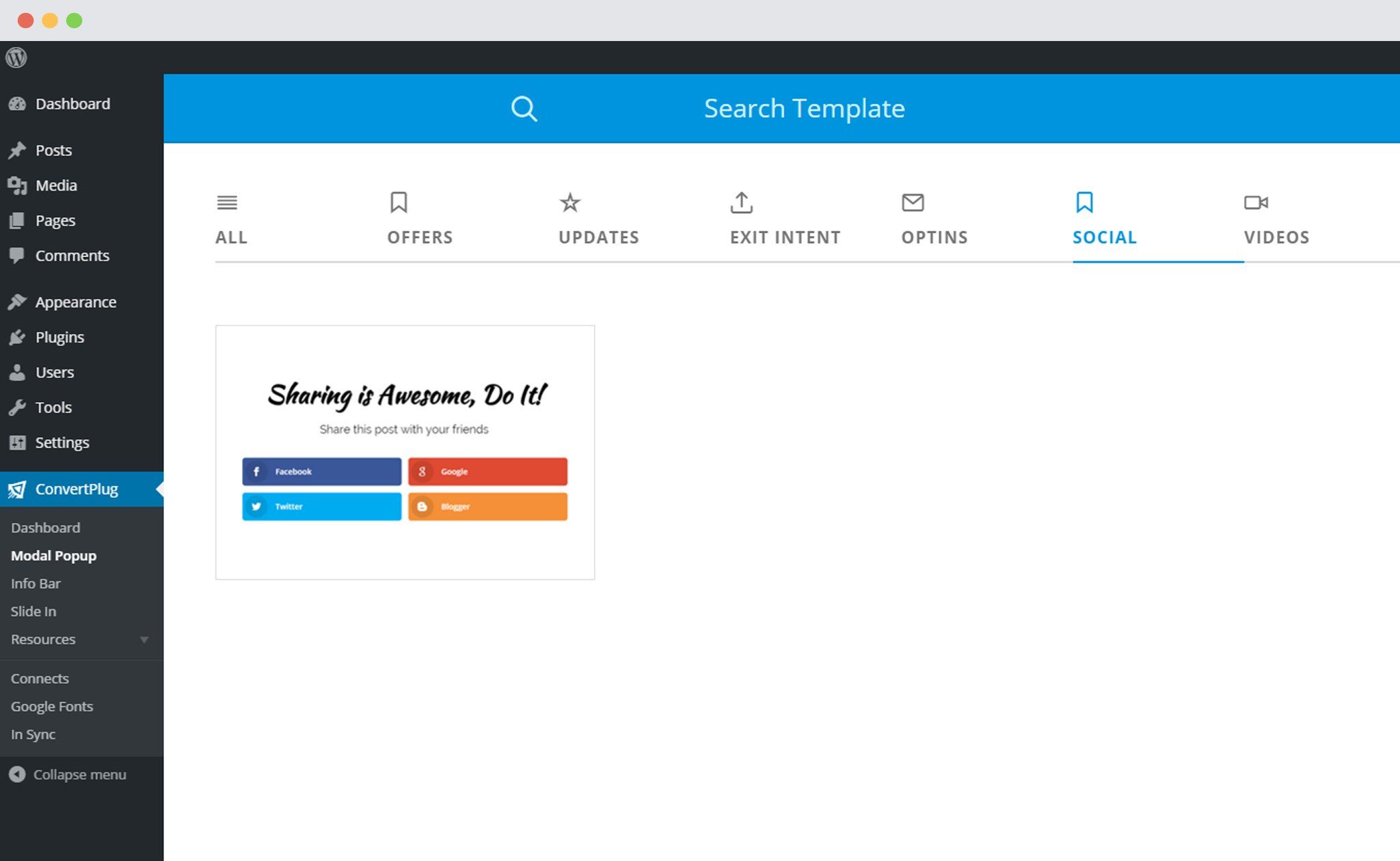This image displays a "Search Templates" page on a computer. At the top of the screen, there's a gray section with red, yellow, and green dots on the left, typical of a macOS window. Below this, a navigation bar begins with a prominent "W" logo, indicating it's a WordPress interface. The sidebar menu on the left shows various options: Dashboard, Posts, Media, Pages, Comments, Appearance, Plugins, Users, Tools, Settings, and ConvertPlug.

The "ConvertPlug" section has been selected, prompting a pop-up message in the center of the screen that reads "Sharing is awesome, do it!" This message encourages the user to share the post with options for Facebook, Google, Twitter, and Blogger. Additionally, the interface displays a menu with options such as Modal Popup, Info Bar, Slide In, and Resources. Other sub-sections include Google Fonts, Integrations, and Sync.

Towards the lower part of the screen, there are tabs labeled All, Offers, Updates, Exit Intent, Opt-ins, Social, and Videos. A search bar is also visible, positioned towards the middle, with a royal blue background highlighting the central area of the page. The overall visual theme and layout suggest an active user interface designed for managing and customizing web content through templates and plugins.